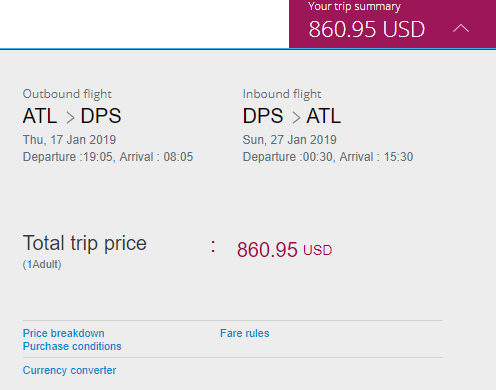This image displays a detailed trip summary, prominently highlighted by the total amount of $860.95 at the top right. Below this, two flight details are presented: 

- On the left, the itinerary shows a flight from Atlanta (ATL) to Denpasar (DPS) scheduled for Thursday, January 17, 2019, with a departure time of 19:05 and an arrival time of 08:05.
- On the right, the return flight details from Denpasar (DPS) to Atlanta (ATL) are shown, scheduled for Sunday, January 27, 2019, with a departure time of 15:30 and an arrival time of 30:15.

The total trip price of $860.95 is repeated in purple text below the flight details. Further down, a price breakdown section and several functional buttons are situated at the bottom of the image, including "Fare Rules," "Purchase Conditions," and "Currency Converter," all presented in light blue. The information is displayed on a light gray background within a rectangular frame, oriented horizontally.